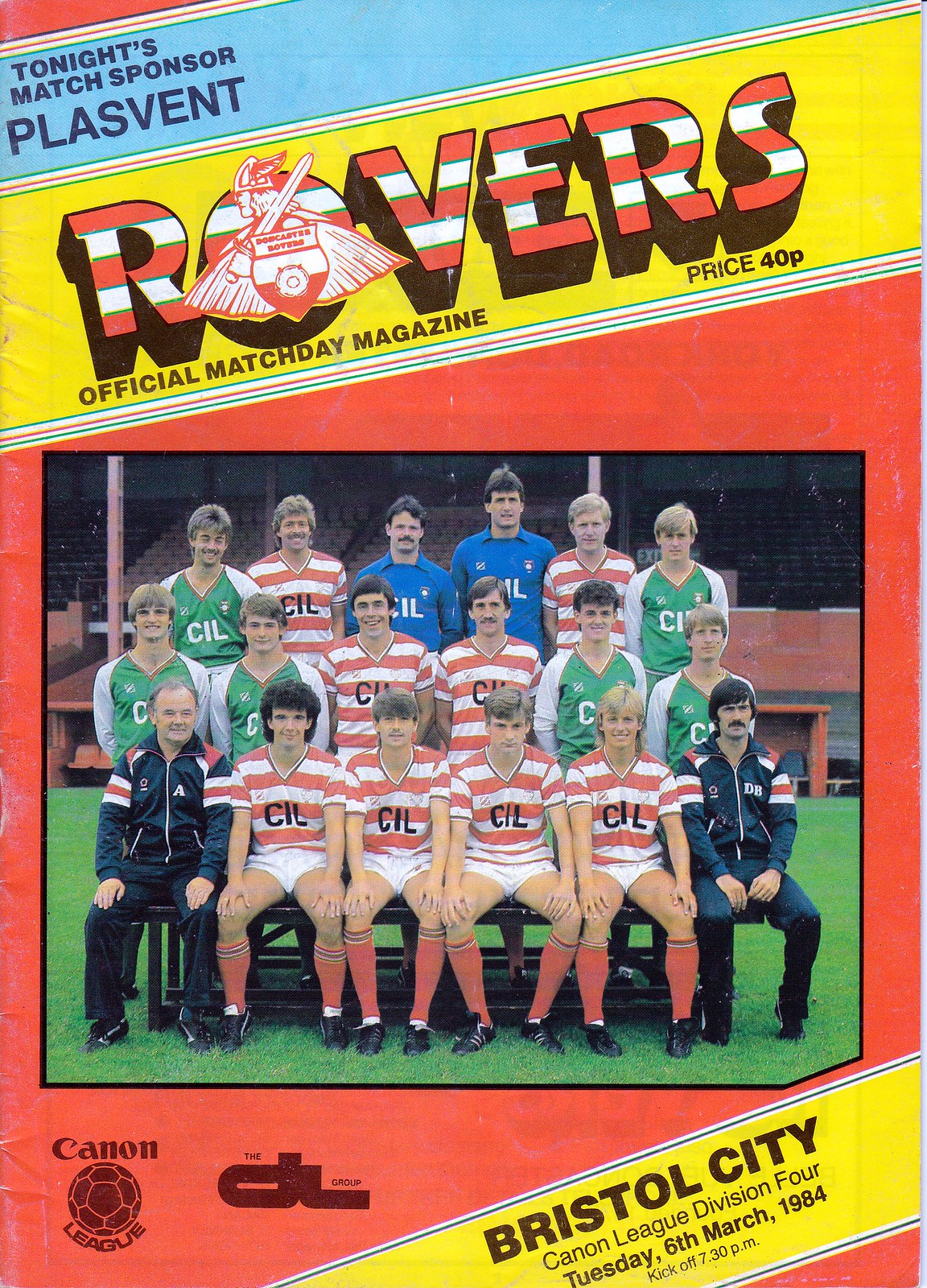This image is the cover of the official match day magazine for Rovers, featuring vividly organized elements and detailed visual contents. At the top left corner, a blue stripe diagonally stretches across, displaying the text "Tonight's Match Sponsor Plazvent" in navy blue font. Below this, a yellow banner prominently showcases the title "ROVERS," written in bold, capitalized letters with red and white horizontal stripes, and a Viking logo embedded in the 'O'. The text "Official Match Day Magazine," along with the price "40p," is printed below the title in a dark color.

The background of the main cover is red, highlighting a large photograph of the Rovers soccer team, posed on a grass field with bleachers visible behind them. The team is arranged in three rows: the front row seated, and the second and third rows standing. Most players wear red and white striped jerseys with white shorts and red socks, while a few wear green jerseys, and two central figures in the back row don royal blue collared shirts. The front row includes two men in navy blue tracksuits with red and white detailing, likely the coaches. At the bottom of the cover, a yellow ribbon runs diagonally across the right-hand side, containing the details "Bristol City Canon League Division 4 Tuesday 6th March 1984, kickoff 7:30 p.m." The Canon League logo featuring the word 'Canon' and a soccer ball underscores the affiliation. This detailed and vibrant cover encapsulates the anticipation and professionalism of Rovers' match day.